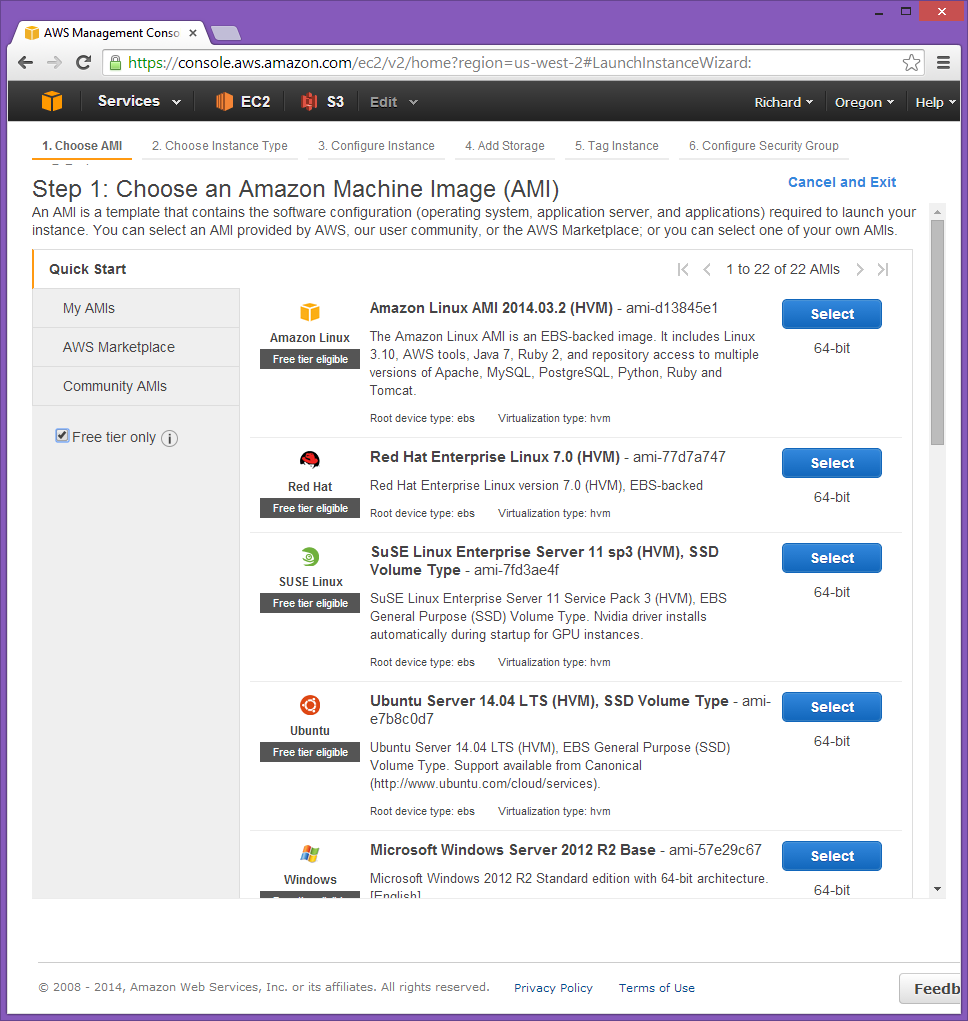The image captures a screenshot from the Amazon Web Services (AWS) Management Console displayed within a web browser. The browser window is in focus with a single tab open, labeled "Amazon Web Services Management Console." The URL is visible in the address bar. 

At the top, there is a thin black navigation bar displaying the AWS logo, a gold-colored cube, and several dropdown menus. The "Services" menu is expanded, showing options like EC2 and S3. To the far right, the bar contains the user's name, Richard, displayed alongside their location, Oregon, and a Help tab. All these elements come with associated dropdown menus.

Below the navigation bar, the main section of the console is shown against a white background. It features six distinct tabs for various setup phases: 1. Choose AMI, 2. Choose Instance Type, 3. Configure Instance, 4. Add Storage, 5. Tag Instance, and 6. Configure Security Group. The active step, "Choose AMI," is highlighted.

On the screen's right side, there is a blue section with options to "Cancel" and "Edit." Below, instructions for step one—choosing an Amazon Machine Image (AMI)—are provided. To the left, different categories for AMIs are listed, including Quick Start, My AMIs, AWS Marketplace, and Community AMIs. A checkbox is available to filter results for free tier AMIs. On the right, a list of available AMIs is displayed.